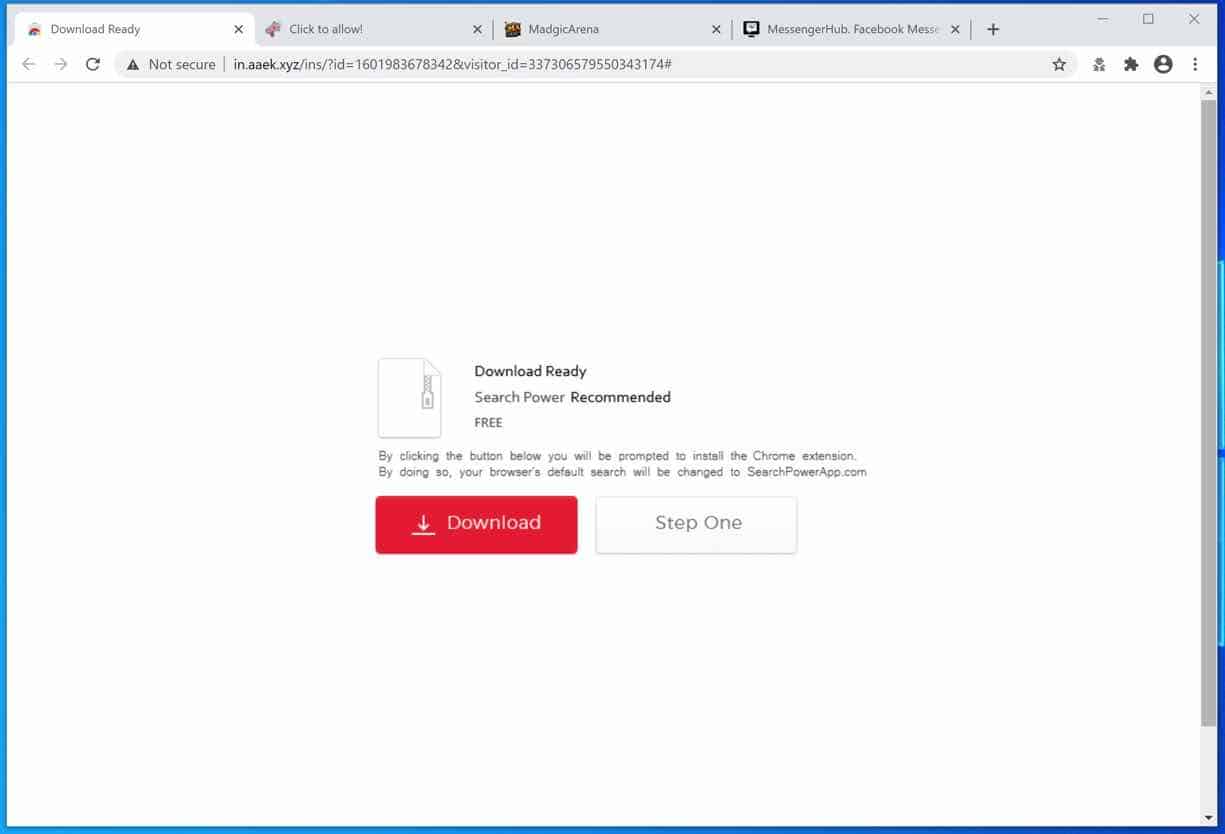The image displays a screenshot of a computer's browser with four open tabs. The tabs, from left to right, are labeled "Download Ready," "Click to Allow," "Magic Arena," and "MessengerHub.FacebookMessin" (with the last label being partially cut off). The active tab shows a web page with an insecure connection, indicated by the URL "Not Secure // in.aaek.xyz" followed by a complex string of numbers and symbols.

The central content of the page features a graphic resembling a paper with a zipper, accompanied by text that states "Download Ready" and "Search Power Recommended." Below that, additional text reads "Free" and explains that by clicking a button, the user will be prompted to install a Chrome extension, which will change their browser's default search engine to "searchpowerapp.com." The page includes a prominent red "Download" button and a smaller white button labeled "Step One."